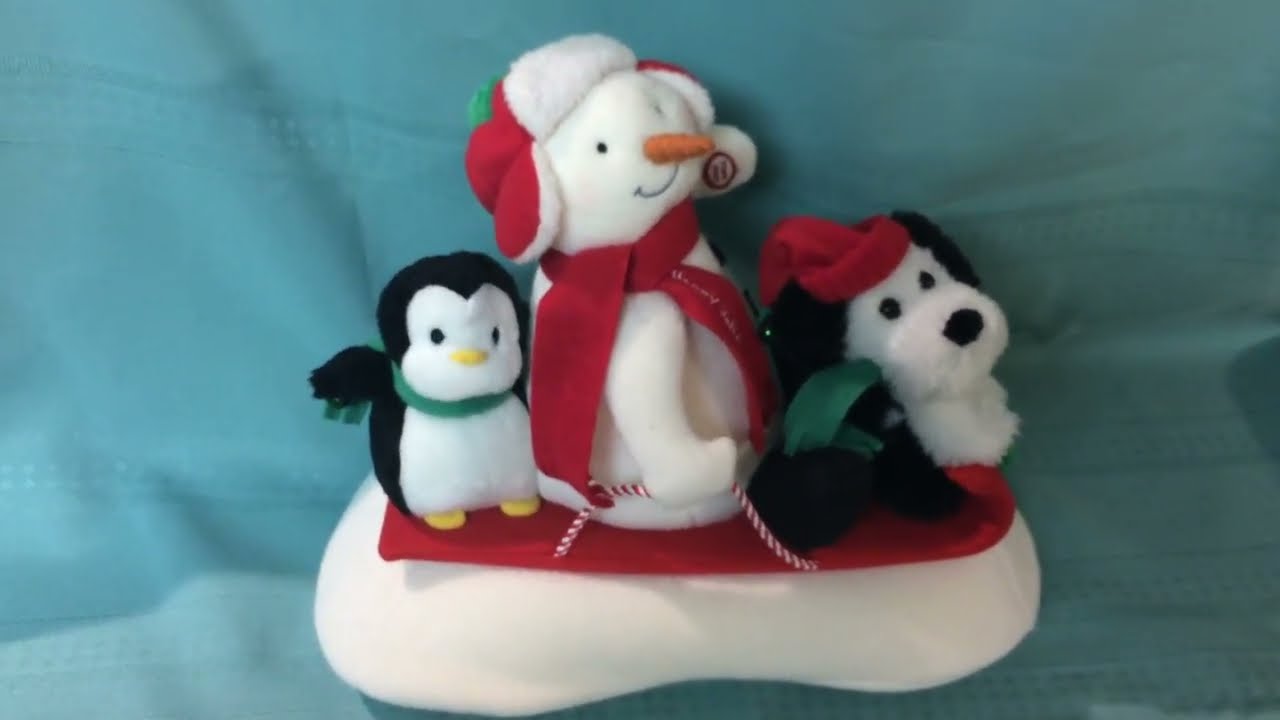The indoor photo features a festive arrangement of three stuffed animals sitting on a red sled atop a white pillow, with a blue or greenish fabric backdrop. From left to right, the stuffed animals include a small black and white penguin wearing a green scarf, a taller white snowman with a carrot nose, a red winter cap, and a red scarf, and a black and white Snoopy-like dog with a white body, black eyes, black nose, and black ears, also sporting a red stocking cap. The snowman, positioned centrally, appears to be holding a red and white striped candy cane rope, adding to the Christmas-themed display. All of the stuffed animals are facing to the right, bathed in festive attire, and collectively evoke a cozy, holiday spirit.